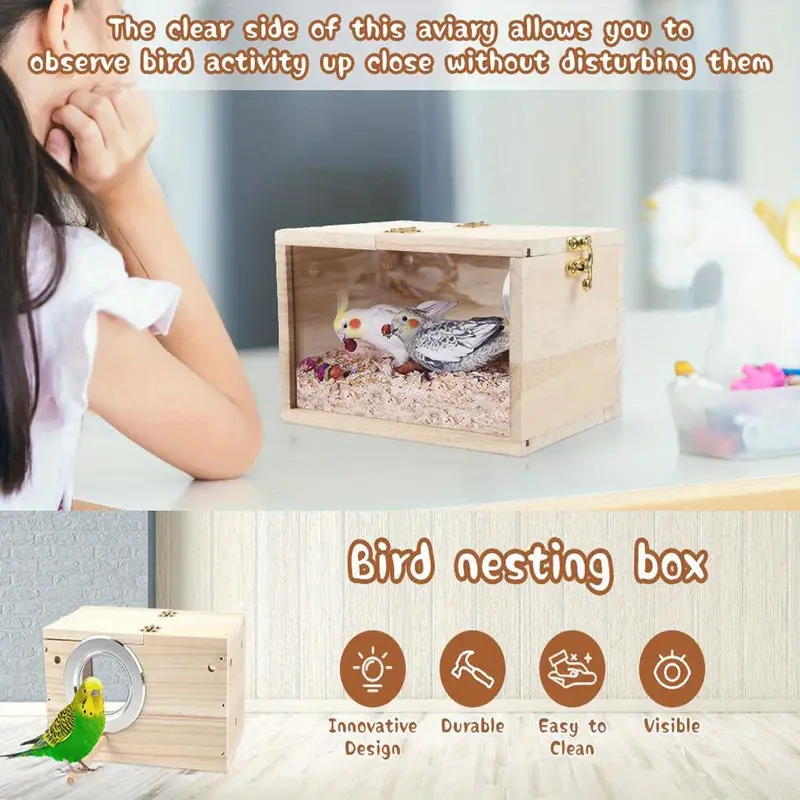The advertisement showcases a bird nesting box with an innovative design that allows for close observation of bird activity without disturbing them. The central image features a young girl with long black hair, wearing a white top, gazing intently at two parakeets inside the light brown wooden box. The box has three wooden sides and one clear plexiglass side, enabling visibility into the avian habitat. The girl, seen from the side, rests her face on one hand and is captivated by the sight of the birds standing on sawdust. The birds, one black-and-white speckled and the other white, appear slightly cramped but active. To the right of the image, there is a small box of bird materials. The bottom of the advertisement highlights the key features of the nesting box with icons: innovative design, durability, ease of cleaning, and visibility. Additionally, a small graphic of another bird nesting box, showing a green and yellow parakeet, is placed in the lower-left corner. The product is depicted as a fun, educational activity for children, with a clear emphasis on its practical and engaging design.